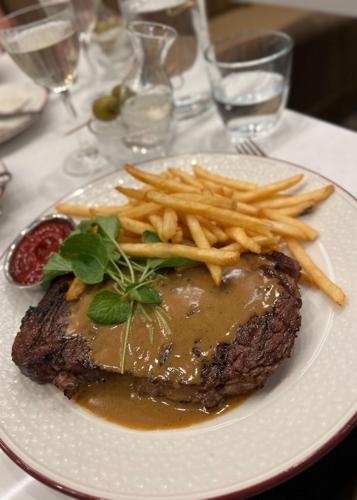The image showcases a dinner setting at a restaurant, featuring a white tablecloth adorned table with a ribbed white plate with a dark red rim. Central to the plate is a well-done steak, enhanced with brown gravy that drizzles to the sides. Topping the steak are light green herbs, adding a touch of freshness. Accompanying the steak is a silver container with a small portion of ketchup, and a generous serving of golden, shoestring-cut french fries. 

To the right of the plate is the partially visible fork. A wine glass and a smaller glass, both filled with a clear liquid that appears to be water, are also seen on the table. Additional visual elements include a container possibly with olives and a large water pitcher in the background. The overall ambiance and the attention to plating details suggest a somewhat upscale dining experience, despite the casual presence of ketchup and fries.